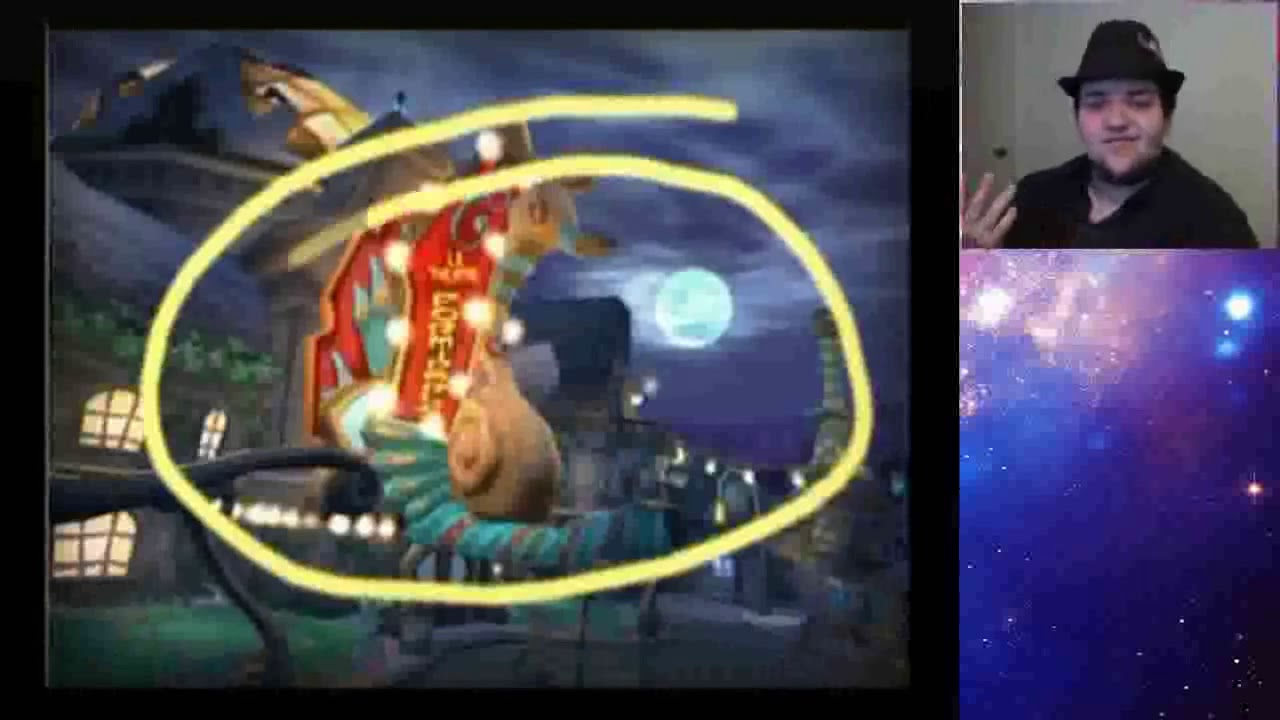The image is an intricate triptych with distinct sections. The left side, occupying approximately three-quarters of the image, features a nighttime screenshot from a video game. The scene centers around a vibrant building adorned with neon lights in red, green, and cream hues, emanating a nostalgic early PS1 graphic quality. Notably, a yellow circular marker highlights the neon sign on this structure. In the background, there's a dark sky with ominous clouds and a full moon emitting a bluish tint.

On the top right corner, there's a small square featuring a selfie of a person with a fair complexion. He wears a black fedora and a black shirt, his patchy beard visible as he raises his right hand to snap the photo. The background behind him is a plain cream-colored wall.

The bottom right section, taking up the remaining area, showcases a cosmic image. This section is filled with an expansive purple and blue galaxy, speckled with stars and nebulae, evoking a sense of the vast universe.